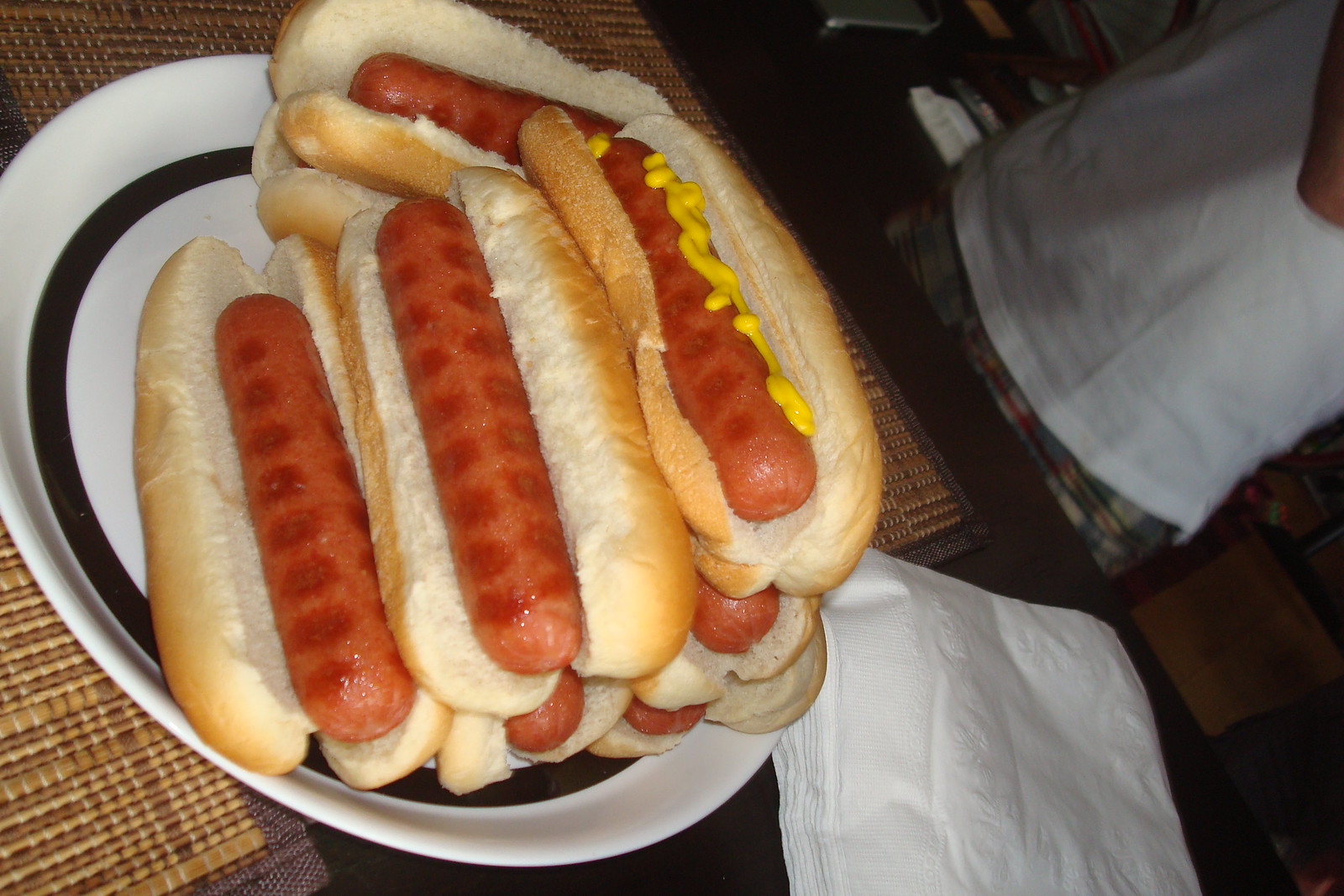This image features a white ceramic plate with a black striped design encircling its inner edge, placed atop a dark brown wooden table with a wicker or teak placemat beneath it. The focal point of the photograph is the plate, which is piled high with approximately eight hot dogs arranged in a pyramid-like formation. These hot dogs are nestled in buns, with one prominently positioned at the top, adorned with a generous squiggle of yellow mustard. The other hot dogs remain plain, devoid of any condiments. In the background, to the right, the torso of a person dressed in a white t-shirt and plaid gray and white bottoms is partially visible, hinting at a kitchen setting. The hot dogs themselves exhibit a peculiar cooking pattern, featuring dark grill spots scattered across their surfaces.